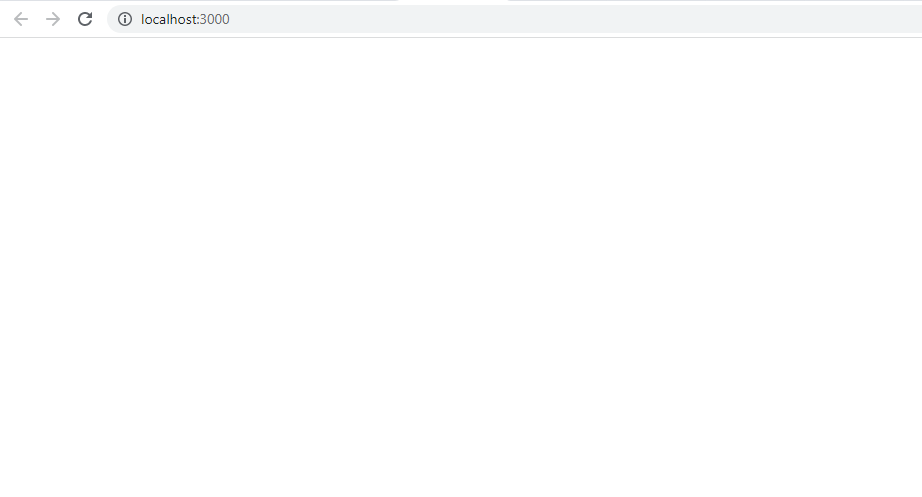The image features a minimalist interface centered around a browser navigation bar. At the very top, there is a thin, horizontal gray line running across the width of the image. Immediately below this line, on the left side, is a back arrow pointing to the left and a forward arrow pointing to the right, both in gray color. Adjacent to these arrows is a reload icon presented with a white background. 

The main element of the interface is a gray search bar. Inside this search bar, towards the left, is an icon of an eye encircled, likely representing an information button. The search bar is displaying the text "localhost:3000" in lowercase. 

Beneath the search bar is another thin, horizontal gray line extending from one side of the image to the other. The overall design is simple, focusing solely on this navigation bar without any additional elements or background distractions.